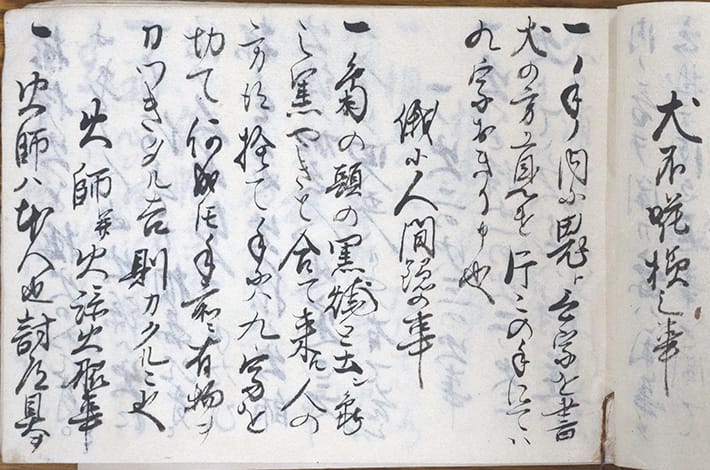This photograph captures an ancient Chinese scroll, meticulously inscribed with bold, black calligraphy characters on thin, aged white paper. The scroll displays 12 vertical lines of characters arranged in a column format. The edges of the paper are tinged with brown, suggesting weathering and age, which adds to the historical allure of the artifact. On the far right of the image, you can partially see the beginning of the next page, indicating the continuation of the script beyond the current scroll. The scroll appears to be spread out, possibly on a wooden surface, with the binding looking worn from frequent use, hinting at its age and the many hands that have perused its contents over time.